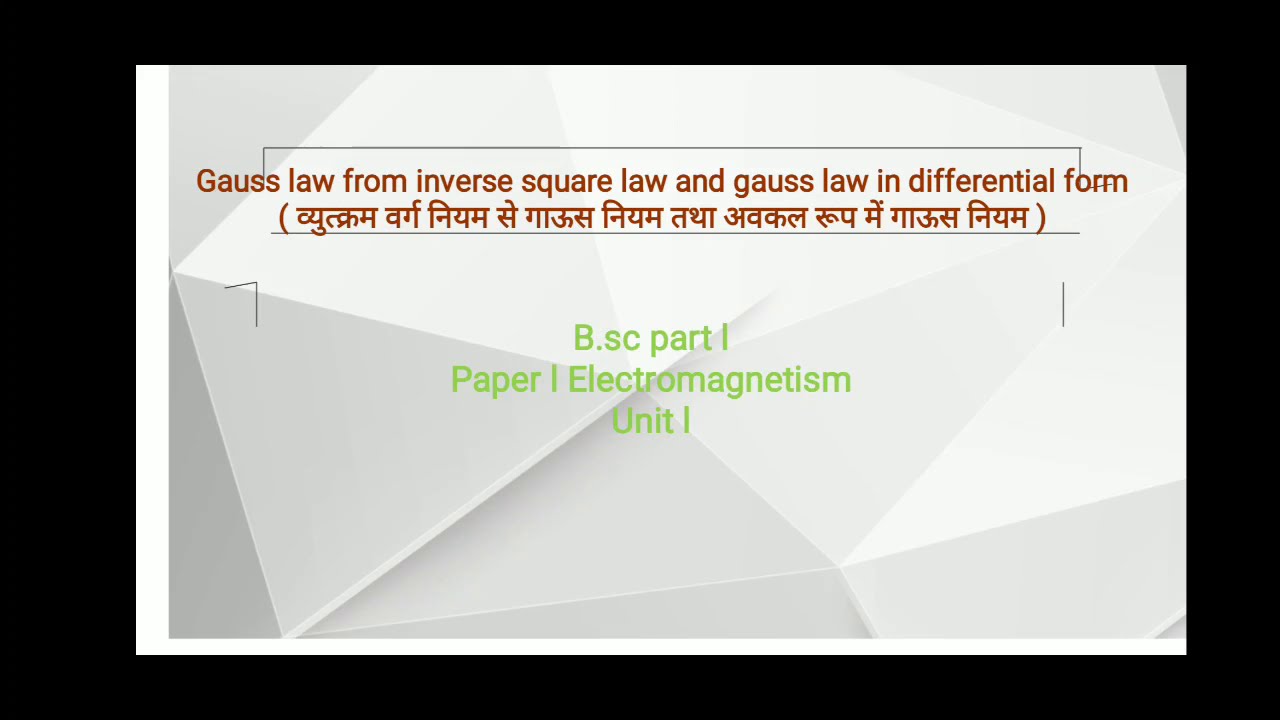The image is a rectangular graphic, possibly a presentation slide or a poster, with a thick black border surrounding a central white area. The background within the white area displays a large light gray and white geometric pattern. There are gradients in the geometric shapes, adding depth to the design. Centrally positioned on the white panel, the main heading is in a dark brown color and reads "Gauss's Law from Inverse Square Law and Gauss's Law in Differential Form." This text is underlined by a line that arcs from the 'S' in 'Gauss' to the 'O' in 'Form'. Directly below this, there is text that appears to be in an Arabic script. Further down, in the middle of the white panel, there are three lines of text in a light green font: "B.SC Part 1," followed by "Paper 1 Electromagnetism," and then "Unit 1." The overall design is suggestive of an educational or scientific topic, particularly focused on electromagnetism and relevant for a B.Sc. course.